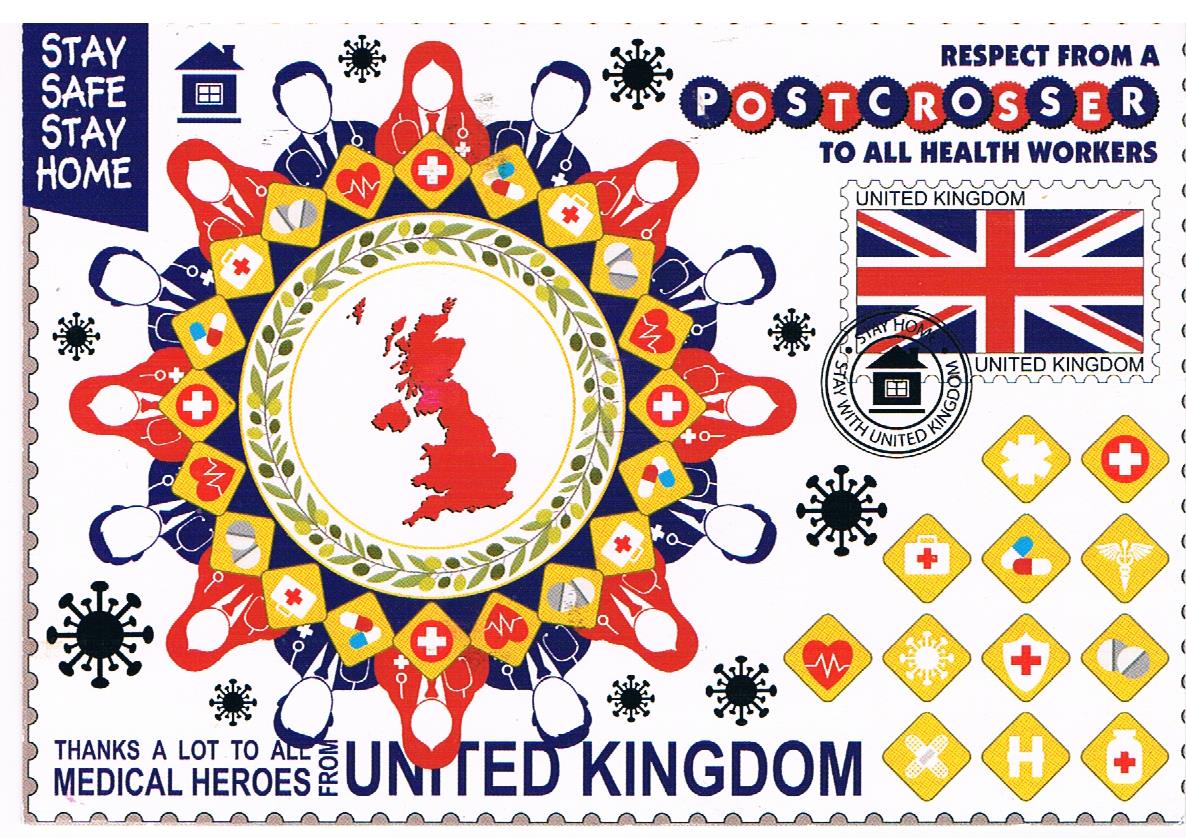The image is a horizontally rectangular, poster-like format, visually reminiscent of a stamp or commemorative card, possibly from the pandemic era. The background is predominantly white. In the upper left corner, there's a blue rectangle with white text that says, "Stay Safe, Stay Home," accompanied by a small house icon. On the upper right, in blue text, it says, "Respect from a post crosser to all health workers," positioned above a small depiction of the United Kingdom flag. Dominating the left side, a large circular seal features a map of England at its center, encircled by green decorative elements and numerous cartoon-like figures of men and women, representing various pandemic workers like doctors, nurses, and other essential personnel. These figures extend around the seal, with some symbols related to their professions. The colors across the image include red, blue, gold, and white, with several icons featuring pandemic-related images scattered throughout. The lower left contains the message, "Thanks a lot to all medical heroes from the United Kingdom," written in blue text. Additionally, there are small black illustrations of coronavirus spike proteins and a yellow square with medical symbols in the bottom right corner.